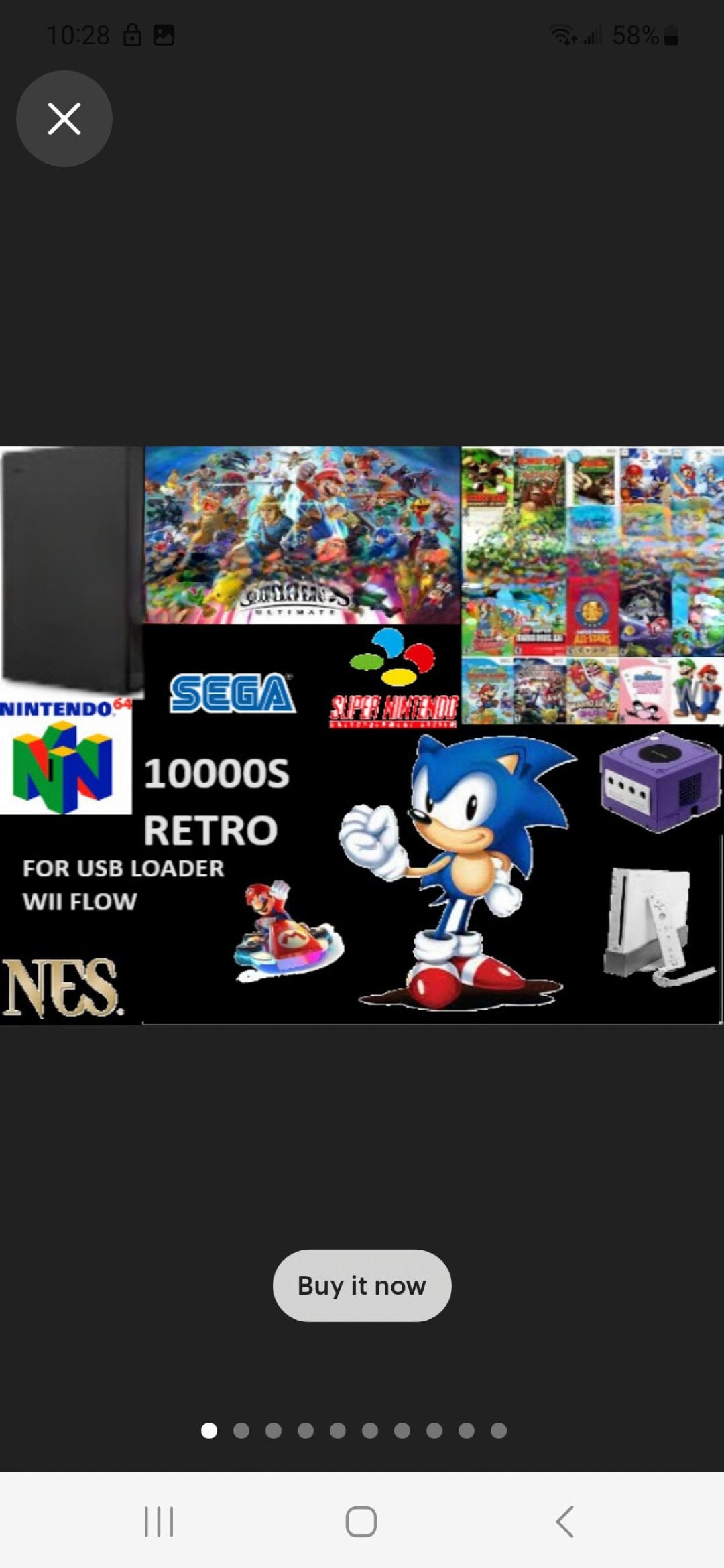The image depicts a person contemplating the purchase of a retro video game emulator system. This device is designed in the shape of classic gaming consoles and promises access to thousands of retro games via a USB loader. Prominently, the console boasts compatibility with multiple classic gaming systems, displaying logos for the Nintendo GameCube, Super Nintendo, Sega, and Nintendo 64.

At the center of the image, a vibrant illustration of Sonic the Hedgehog takes the spotlight. Sonic is depicted with his signature blue spiky hair, white gloves, and red shoes, striking a dynamic pose with his fist clenched in the air. Below the Sega logo, there is a smaller emblem featuring Mario riding a Mario Kart.

Text on the console highlights "10,000 Retro" games available, with the phrase "for USB loader wifi flow" written in smaller font beneath it. In the bottom left corner, the NES logo is visible, while the top left corner features a large 'X'. There is an indistinct background element behind the 'X', possibly indicating battery life at 58%, although the text is quite faint.

At the bottom center of the image, a prominent "Buy Now" button is displayed in white. Adjacent to this button, a series of nine or ten dots suggests the presence of additional images or features for the viewer to browse. Below these dots, three vertical lines are positioned to the left, with a square in the center and a left arrow to the right, indicating possible navigation controls.